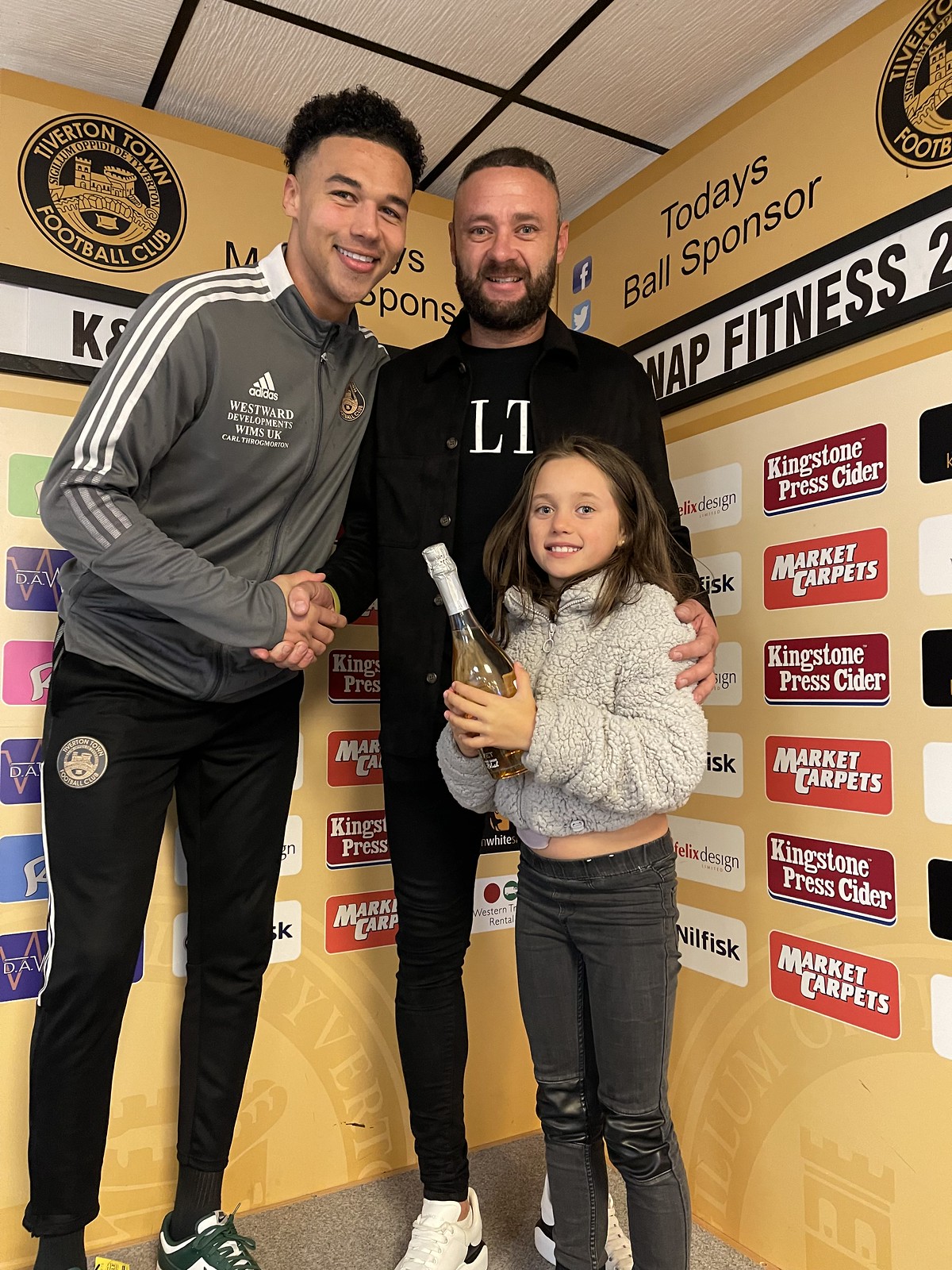In this color photograph with a portrait orientation, three individuals—a young girl and two men—are posing for a picture with smiles on their faces. They are standing in front of a yellow wall adorned with multiple rectangular signs that advertise sponsors. Among these signs, you can clearly read "Today's Ball Sponsor" and "WAP Fitness." Additionally, the text mentions "Kingston Press Cider Market Carpets" repeated several times in alternating red and lighter red colors.

On the far left stands a man who appears to be about 22 years old. He is wearing a gray track jacket with a white insignia on the right breast, dark pants, and sneakers. He is in the middle of shaking hands with the second man, who stands to the right. This second man, estimated to be between 35 to 40 years old, sports a LT visible on his black T-shirt, a darker athletic jacket, dark jeans, and light sneakers. 

Occupying the center and standing in front of these two men is a young girl, around 10 years old. She holds a bottle that resembles champagne or wine and is dressed in a fuzzy gray sweater and dark leather jeans with patches. Her dark shoulder-length hair frames her face as she beams at the camera. 

Behind this group, on the top left of the image, there's a round logo bearing the name Tiverton Town Football Club with gold lettering circling the edge. This detailed and vivid scene captures the essence of a cheerful moment shared among soccer enthusiasts and sponsors.